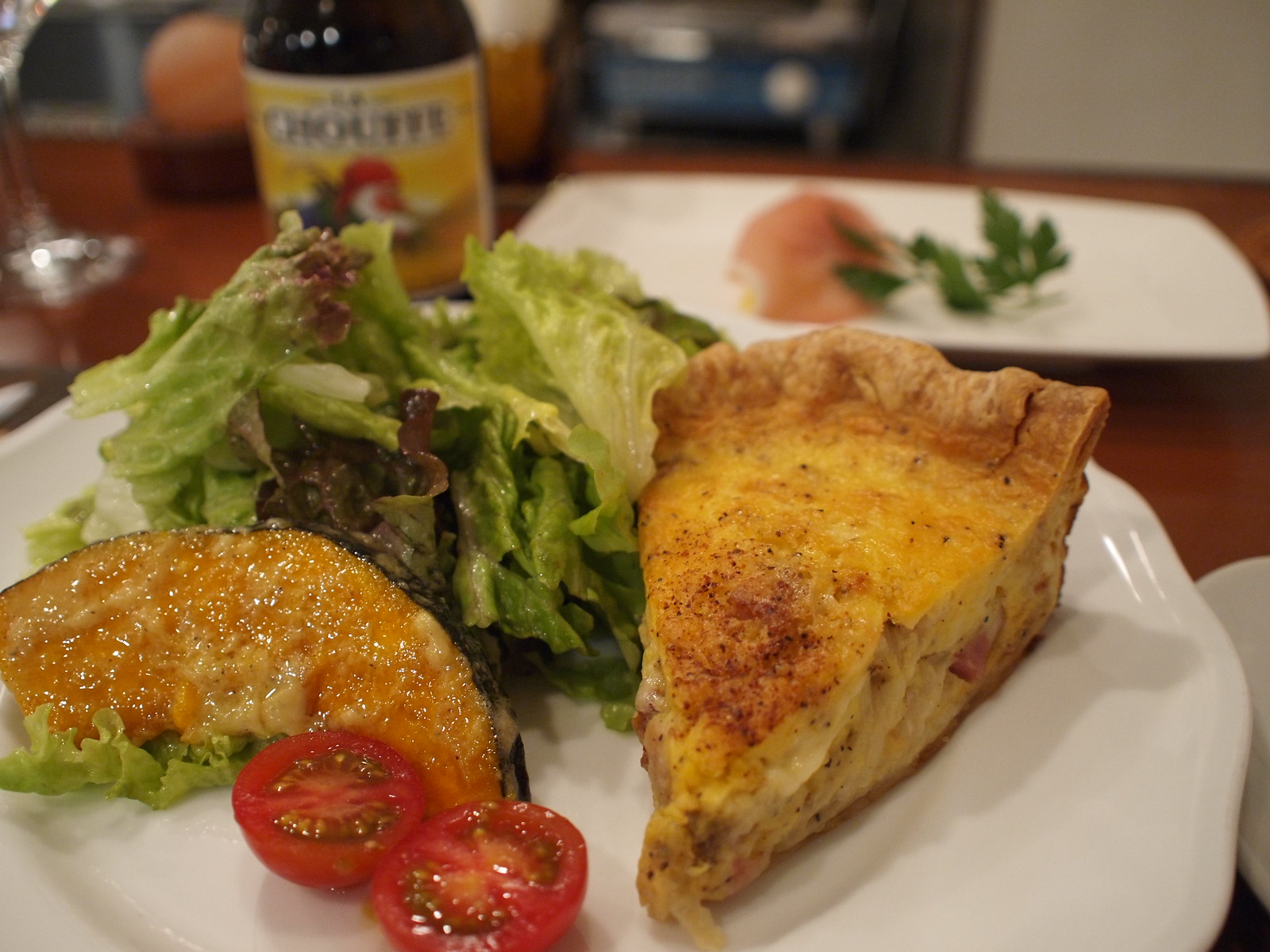The image depicts an indoor scene at a fancy Italian restaurant. On the table, which is brown, there is a variety of food artistically presented on white plates. The foreground plate features a small salad with lettuce at the top, a half-moon shaped item with a dark crust and orange middle, and a cherry tomato cut in half. To the right on the same plate, there is a slice of quiche, golden-yellow on top with visible eggs and ham. In the background, on another white plate, there's garlic bread and another type of bread covered in butter, along with additional salad components. A fancy beer bottle can be seen in the background, slightly blurred, accompanied by a glass of wine to the left along with some empty wine glasses. The overall setting, enhanced by a white wall behind the table, reflects the elegance and sophistication of a high-end Italian dining experience.